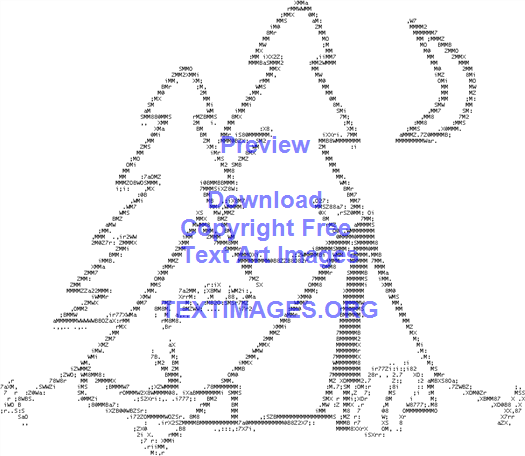The image is a computer-generated, black-and-white illustration with a white background. Dominating the scene is a large Christmas tree with jagged branches positioned in the middle. A tent, slightly covering the base of the central tree, is pitched in the foreground. Next to this central tree, toward the left, is another tree of similar design. Up in the top right corner, a crescent moon suggests a nighttime setting despite the white backdrop. The composition is made using an assembly of numbers and dots, giving it a simplistic yet intentional appearance. In the center of the image, prominently displayed in blue lettering, are the words "Preview" followed by "Download Copyright-Free Text or Images," with the URL "textimages.org" below. This gives the impression of a printout, akin to an image printed on standard black-and-white printer paper. Additionally, subtle details like someone's feet protruding from the tent add a human element to the scene.